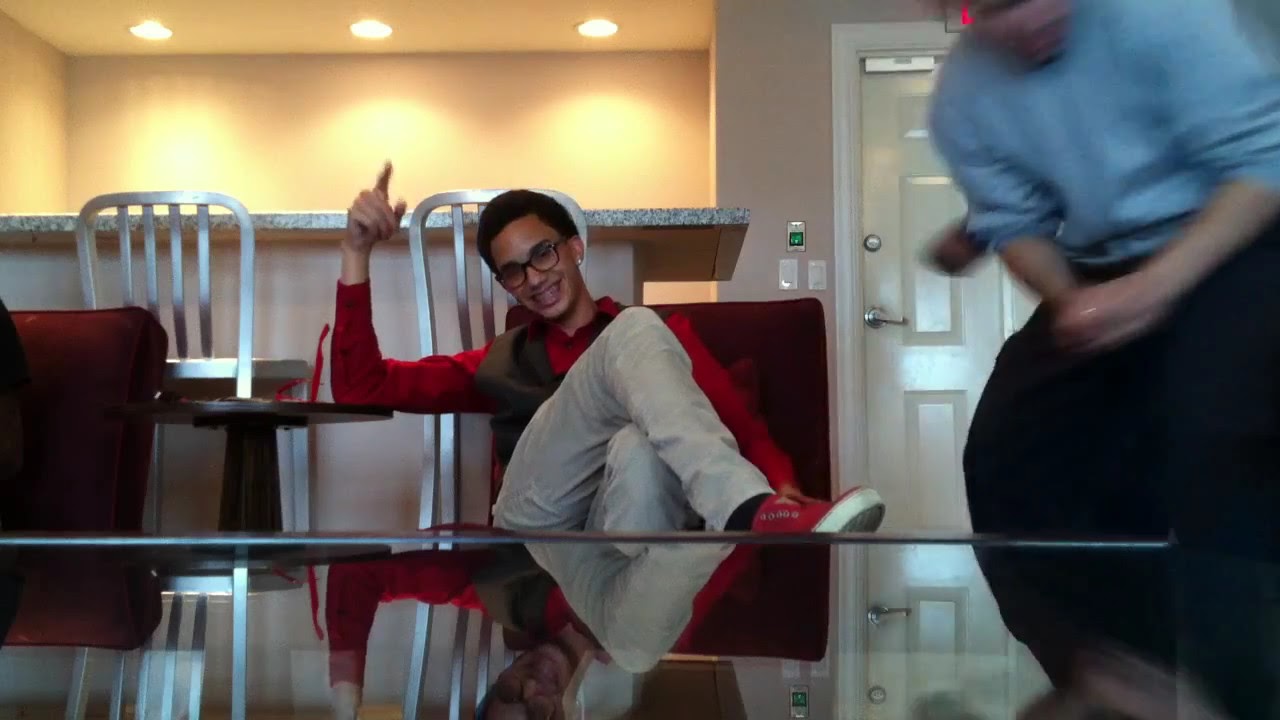In a warmly lit room, two men are present. At the center is a gentleman with short, dark hair, slightly dark skin, and glasses, sitting comfortably on a red chair. He wears beige pants, a red shirt, a dark vest, and bright red shoes. His legs are crossed, one hand is resting on a nearby table, and he is holding one finger in the air while smiling broadly. Notably, the table in front of him creates a reflective surface, mirroring the upper part of the scene. To his right, slightly blurred, stands another man dressed in a blue shirt and black pants, who appears to be slightly hunched over. The background features a high counter area with two high counter stools, overhead recessed lighting, and a door with visible latches. The room's overall ambiance is further enhanced by the presence of a small table with two red chairs, contributing to its cozy atmosphere.